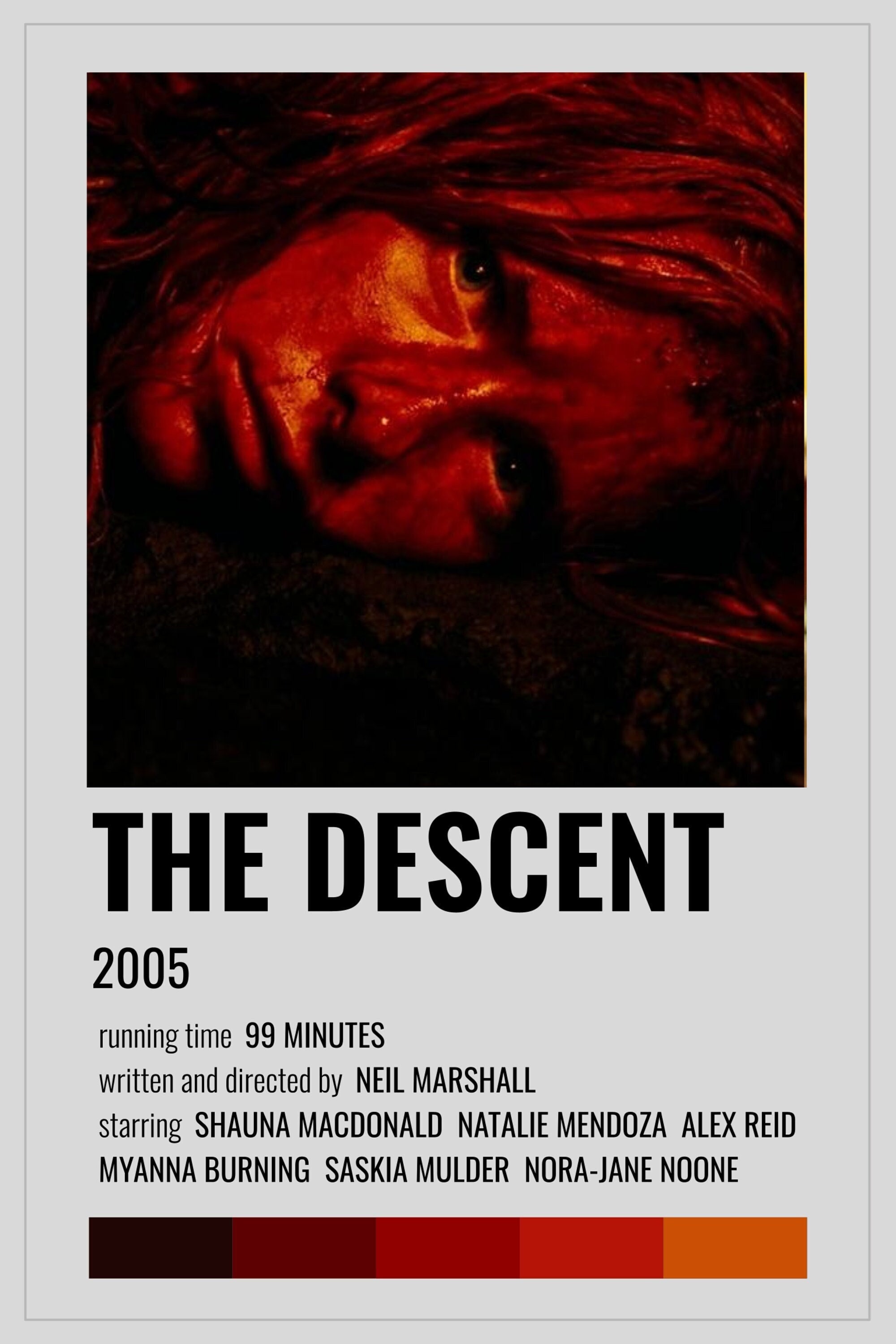The image resembles a movie poster with a light gray background. Dominating the top half is a striking picture of a woman's face turned sideways, drenched in red, possibly blood. The expression on her face is one of intense fear. Below this haunting image, the title "The Descent" is displayed in bold black font, followed by essential details: "2005, running time 99 minutes, written and directed by Neil Marshall," and the cast list, "starring Shauna MacDonald, Natalie Mendoza, Alex Reid, MyAnna Buring, Saskia Mulder, and Nora-Jane Noone." Beneath the text is a gradient line transitioning from dark burgundy to wine red, blood red, and finally to orange. This detailed composition appears to be a printed scan or a graphic design mock-up rather than an actual physical poster.